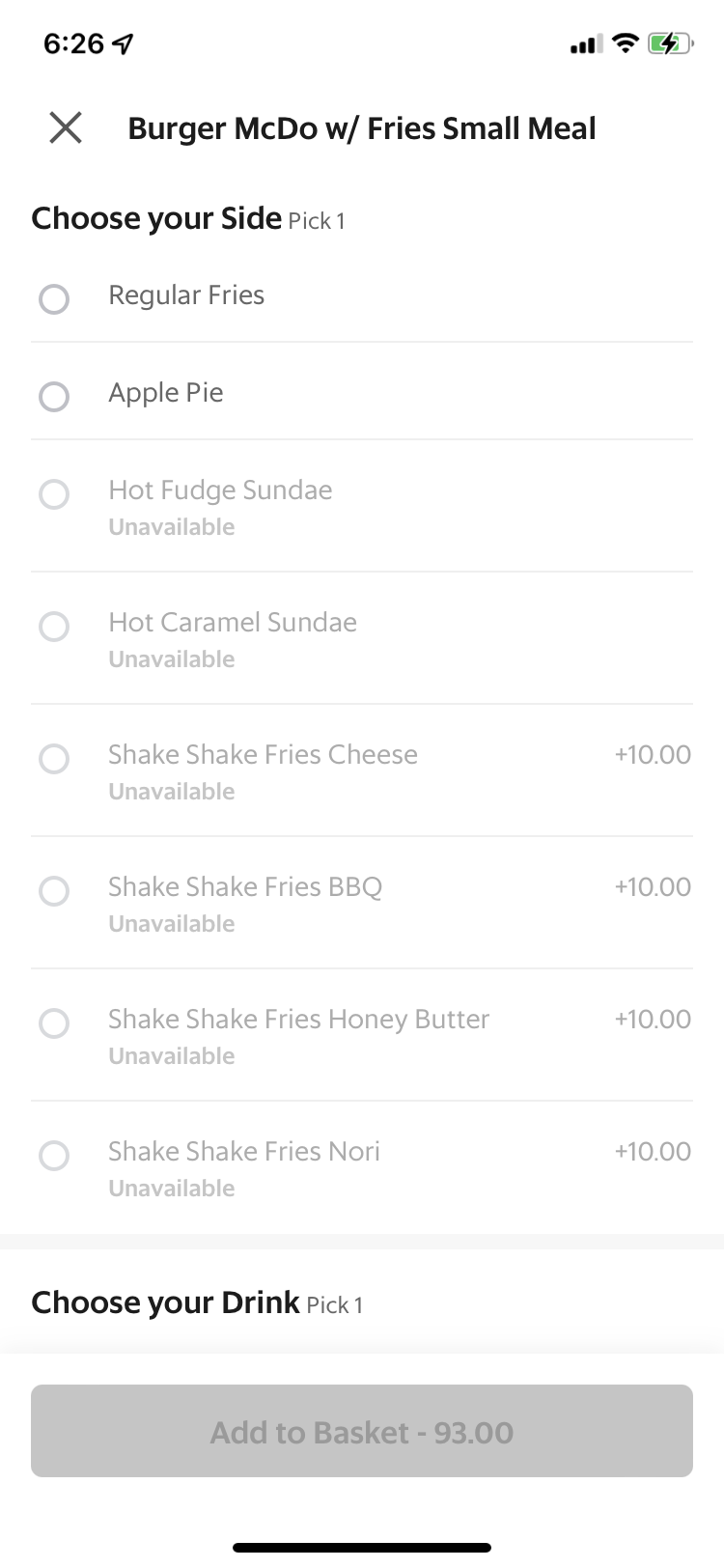The image displays a screenshot from an Apple mobile device, showing the interface of what appears to be a McDonald's ordering app. The device status bar indicates it's 6:26 AM, with location services active, 3 out of 4 bars for cellular connection, full Wi-Fi signal, and approximately 75% battery charge. 

At the bottom of the screen, a black line suggests the option to minimize or close the app. The top portion of the screenshot features a black 'X' button and black text reading "Burger McDo with fries, small meal," likely indicating the McDonald's Burger McDo meal offering. 

The interface prompts the user to choose a side, although most options are unavailable and grayed out, except for "Regular Fries" and "Apple Pie." Detailed prices are visible for several unavailable sides, including various "Shake Shake Fries" flavors (Cheese, Barbecue, Honey Butter, Nori), each priced at $10. 

This limited availability and the unusual side options suggest a non-U.S. location, possibly with localized menu items. At the very bottom of the screen, the user is asked to choose a drink and make a final selection to "add to basket," although this option is currently grayed out and marked with the number "93."

In summary, the screenshot captures someone navigating a McDonald's ordering app, likely outside the United States, trying to assemble a meal with limited side options and grayed-out selections.